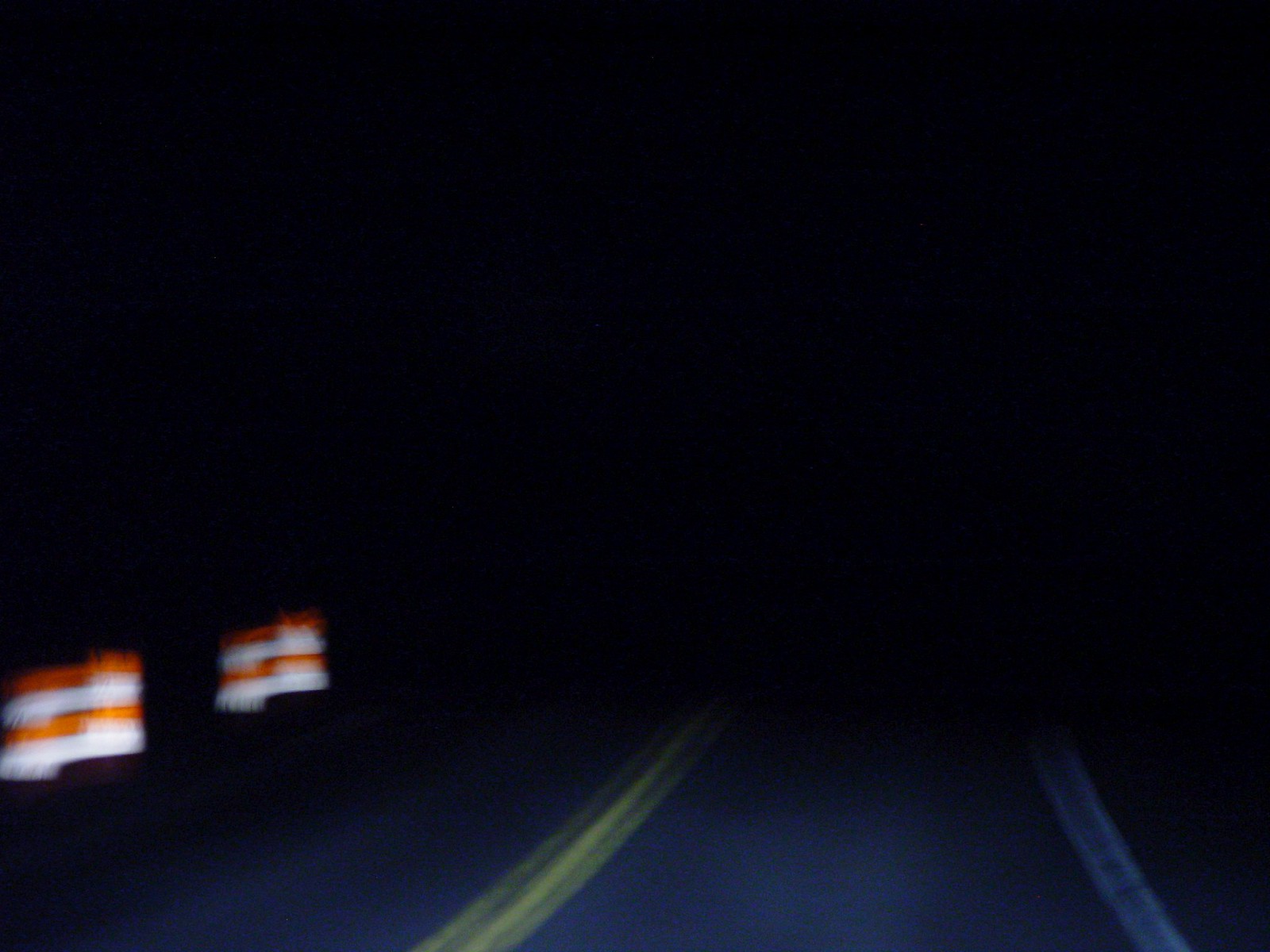The image is a dark, blurry view from a vehicle, likely taken through the windshield at night. It captures a two-lane road with the lanes separated by a solid yellow line. The right-hand side of the road features a blurry white line marking the shoulder. The road is dimly illuminated by the vehicle’s headlights, barely piercing the pitch-dark surroundings. On the left-hand side, near the bottom of the image, there are two orange and white striped barriers or construction drums, potentially serving as a cautionary warning to the driver. The top two-thirds of the image fades into complete darkness, emphasizing the limited visibility and nighttime setting.